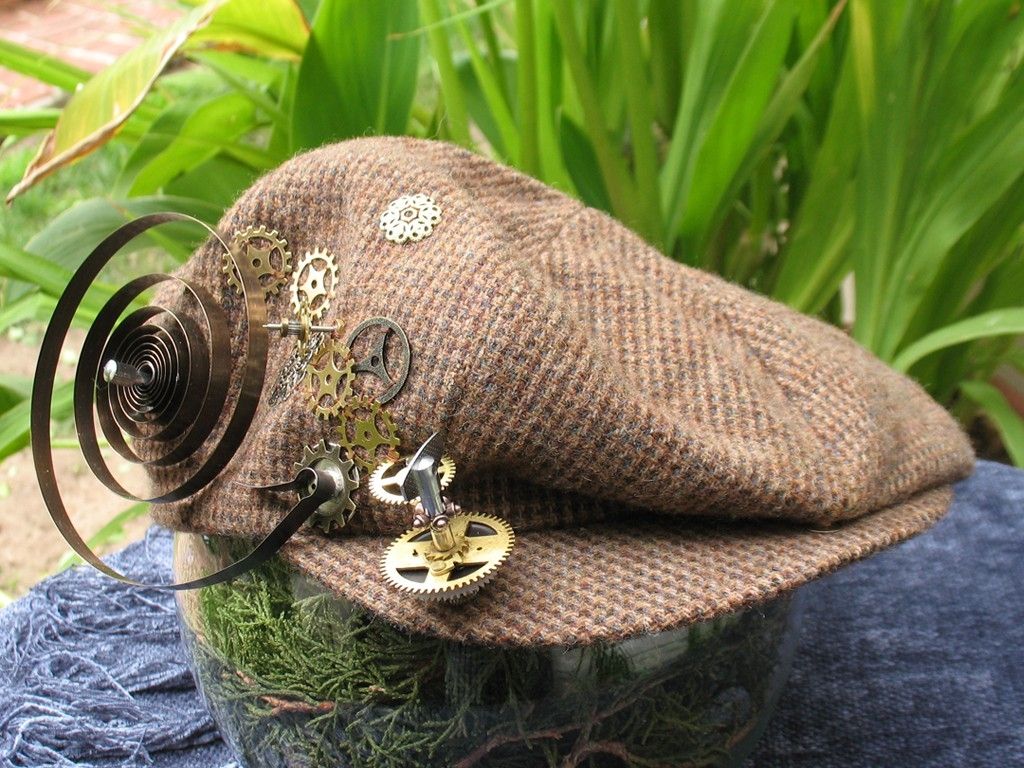This close-up image features a brown tweed slouch hat, adorned in a steampunk fashion with a variety of metallic elements. The hat is decorated with an assortment of gears—some in gold and black hues—and a white flower-like pin. A long, coiled copper wire extends from the hat’s bill, adding to its intricate design. The hat is positioned atop a transparent glass vessel, which sits on a denim-like blue fabric, possibly yarn. The background is filled with lush green foliage, resembling tall grasses or possibly tulips or irises, adding a natural contrast to the mechanical aesthetic of the hat. The entire scene is set on a rock, with grey material visible on its side, giving the image a blend of rustic and industrial vibes.